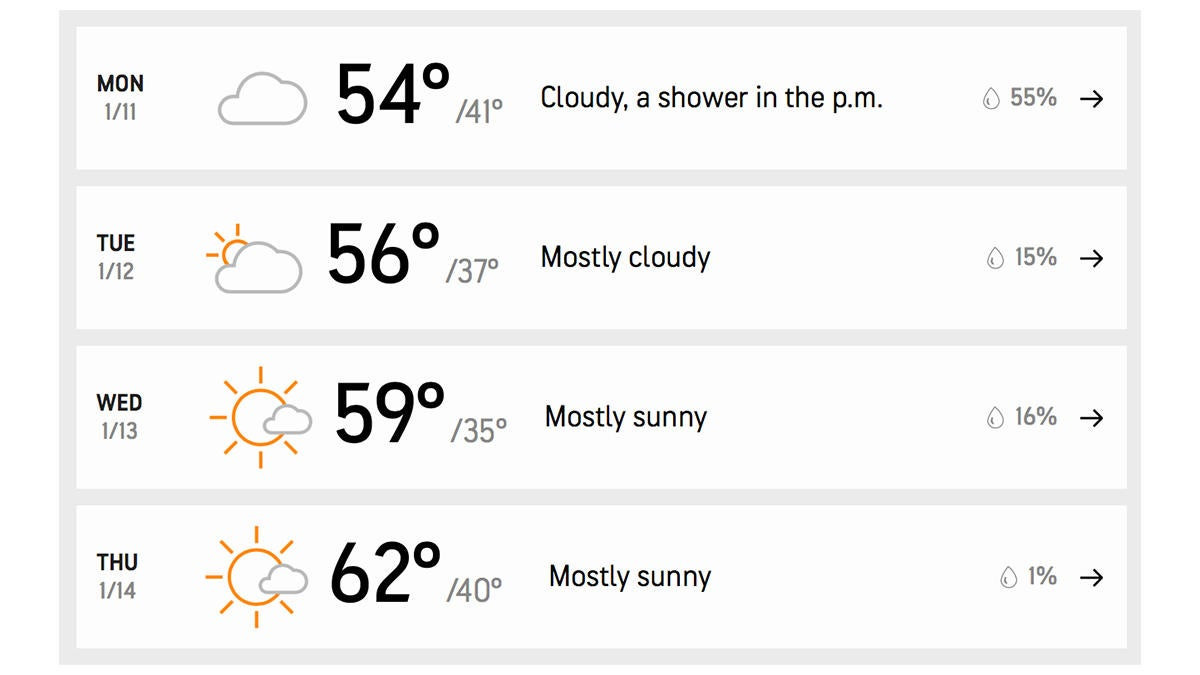This screenshot from a weather application, taken from an unspecified mobile device, showcases a detailed four-day weather forecast. The user interface consists of four elongated, rectangular panels set against a light gray-pinkish background. Each white panel is methodically structured with the following details:

1. **Monday, January 11th**:
   - Weather Icon: Cloudy
   - Temperature: High of 54°F / Low of 41°F
   - Description: Cloudy with a shower in the PM
   - Chance of Rain: 55%

2. **Tuesday, January 12th**:
   - Weather Icon: Partly Cloudy
   - Temperature: High of 56°F / Low of 37°F
   - Description: Mostly cloudy
   - Chance of Rain: 15%

3. **Wednesday, January 13th**:
   - Weather Icon: Partly Cloudy, Mostly Sunny
   - Temperature: High of 59°F / Low of 35°F
   - Description: Mostly sunny
   - Chance of Rain: 16%

4. **Thursday, January 14th**:
   - Weather Icon: Partly Cloudy, Mostly Sunny
   - Temperature: High of 62°F / Low of 40°F
   - Description: Mostly sunny
   - Chance of Rain: 1%

The information provided focuses on day-by-day weather conditions, temperature ranges, brief descriptions of the weather, and the percentage chance of rain for each day, aiding in a comprehensive understanding of the upcoming weather trends.